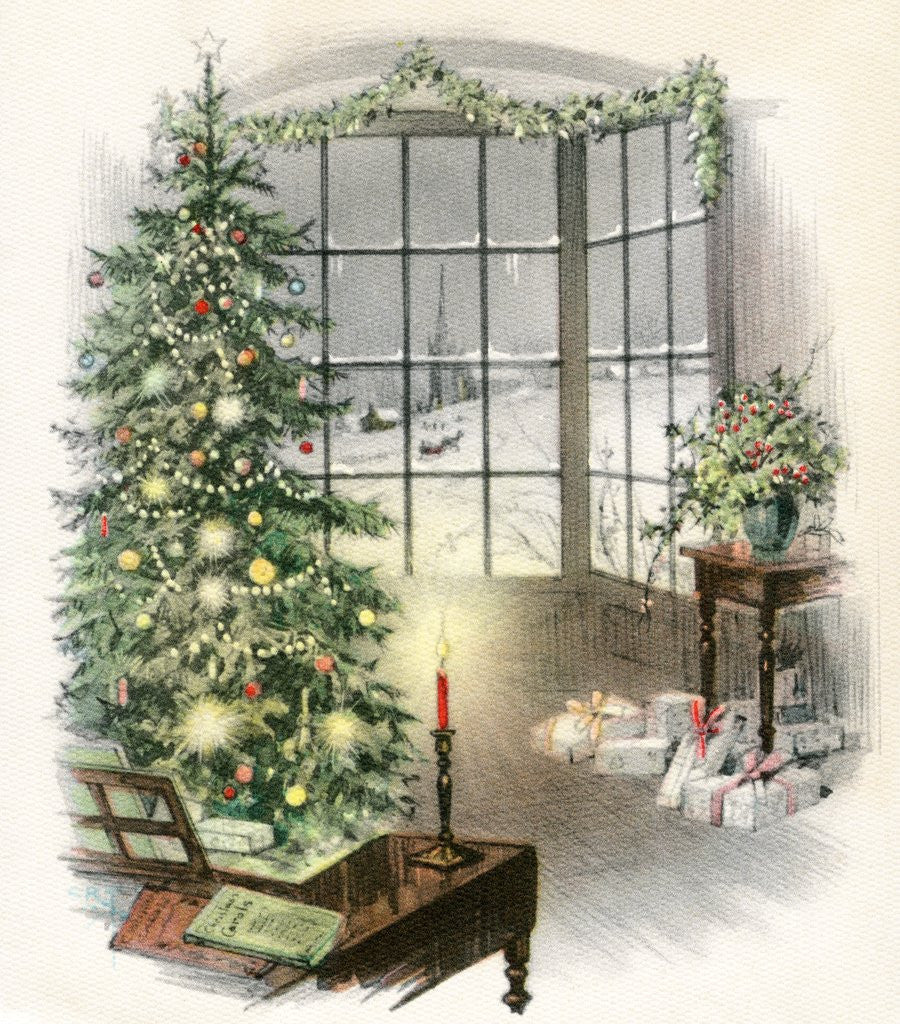This artist's drawing, evocative of an old-fashioned Christmas postcard, depicts a cozy indoor holiday scene. Dominating the left-hand side of the image is a magnificent, decorated Christmas tree adorned with colorful ornaments. Adjacent to the tree, there is what appears to be a piano, suggested by the presence of sheet music and a red tapered candle on its surface. A book titled "Christmas Carol" further supports the piano's presence. 

In the background, a large panelled window reveals a serene, snow-dusted landscape. Through the window, snow falls gently, blanketing the ground and the rooftops of distant houses. A church spire rises prominently amidst the snowy skyline, adding a touch of tranquility to the scene. 

To the right of the window stands a wooden side table bearing a vase with Holly and Ivy. Beneath this table, several presents wrapped in pink and red bows are carefully arranged. Another smaller stand near the Christmas tree holds a pot with a plant, adding to the festive decorations. The entire setting exudes warmth and nostalgia, making it a perfect illustration for a Christmas card.